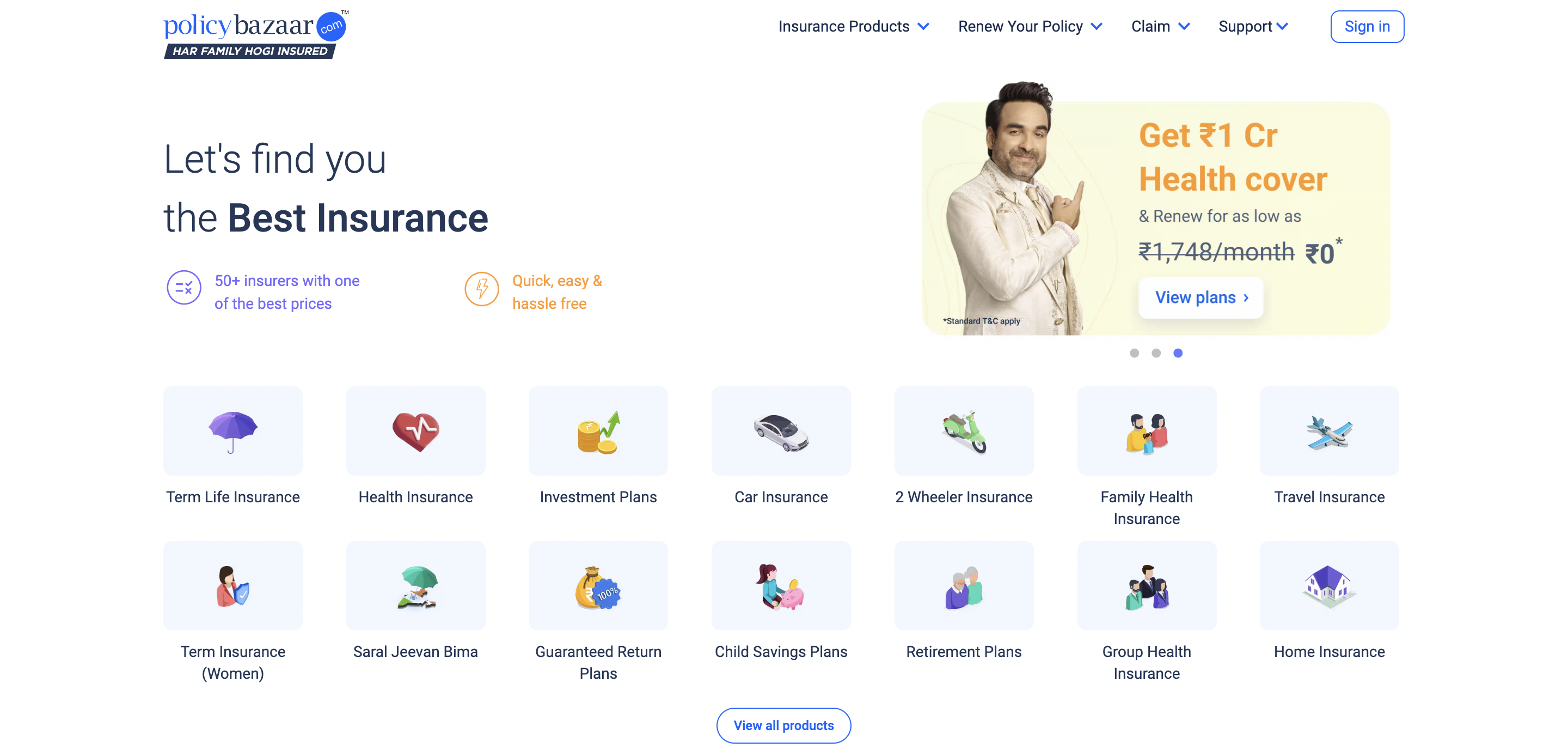This is a detailed screenshot from the website Policy Bazaar. At the top of the page, there's a banner with the text "Har Family Hodge Insured" prominently displayed. The website's title, "Policy Bazaar," is written in blue, with ".com" enclosed in a blue bubble. 

On the left side, the title of the website reads, "Let's find you the best insurance," while on the same row to the right, there's an advertisement featuring a man in a cream suit. The ad contains orange text stating "Get $1 Health Cover," and features a blue bubble with the text "View Plans."

Below this, there are two rows of icons, each representing different sections of the website. The first row includes:
1. **Term Life Insurance** - represented by a purple umbrella.
2. **Health Insurance** - depicted as a heart with a line through the middle.
3. **Investment Plans** - shown as a stack of gold coins with a green upward arrow.
4. **Car Insurance** - illustrated by an image of a silver car with a black roof.
5. **Two-Wheeler Insurance** - symbolized by a green moped.
6. **Family Health Insurance** - depicted by three figures: a husband, a wife, and their child.
7. **Travel Insurance** - represented by an airplane.

The second row, from left to right, features:
1. **Term Insurance** - illustrated by a woman in a pink suit.
2. **Saral Jeevan Bima** - symbolized by a person on a moped holding up a teal umbrella.
3. **Guaranteed Return** - shown as a money bag with a prize icon labeled "100."
4. **Child Savings Plan** - depicted by a mother taking care of a child.
5. **Retirement Plans** - represented by an elderly couple.
6. **Group Health Insurance** - illustrated by three people dressed in business suits.
7. **Home Insurance** - symbolized by a house with a purple roof.

At the bottom center of this section, there is a blue bubble with the text "View All Products."